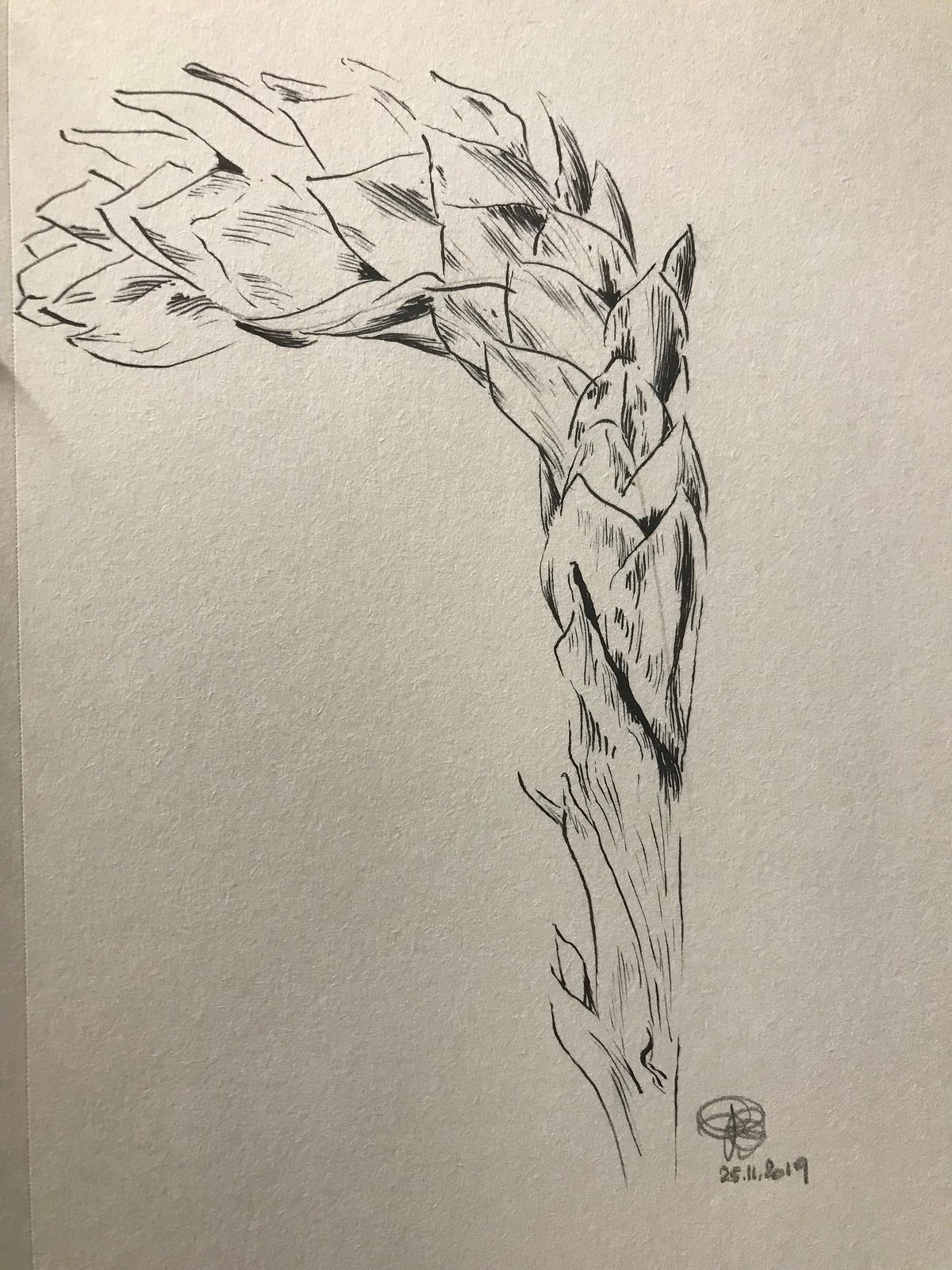The image is a detailed, monochromatic drawing, rendered in either black pen or ink, on a light sandy brown or pale gray piece of paper. The background provides a neutral canvas that enhances the intricate shading and textures of the subject. Starting from the slender, faded base of the plant, the stem rises upwards with visible wood fibers. As it ascends, it gradually gains definition, eventually curving gracefully to the left. The drawing evokes the structure of a plant or tree with a stark resemblance to an upside-down palm or coconut tree trunk, characterized by an array of interlocking, artichoke-like leaves that create a complex, layered appearance. The top of the plant fans out more broadly than the lower sections, adding to the illusion of weight at the apex, causing a subtle bend to the side. The bottom right corner is marked by the artist's signature and a date, partially legible as "25.11.2019," subtly indicating the artwork's creation date.